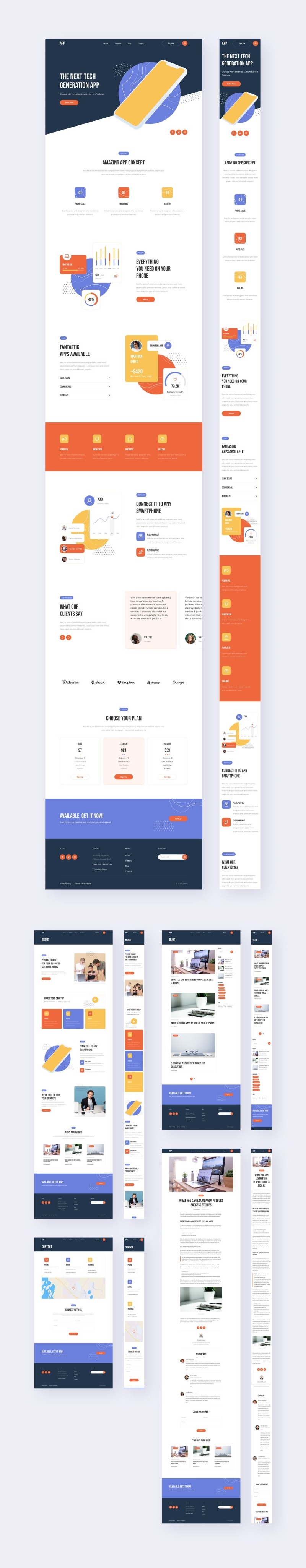The vertical image showcases a series of different webpages designed for a smartphone device. Despite their variety, these pages share a consistent aesthetic with a gray background and a prominent white header displaying the word "App." At the top-right corner, an eye-catching orange button stands out. 

Central to the design is an icon featuring a white iPhone with an orange interface, positioned against a purple circular backdrop. The title "Next Tech Generation App" is prominently displayed, followed by the description "Amazing App Concept." Several interactive elements are presented, such as clickable tabs for different steps: Step 1 in purple, Step 2 in orange, and Step 3 in yellow. These sections also feature informative charts and percentages, emphasizing the app's practical benefits.

Additional notes include assertions of the app's versatility, suggesting "Fantastic apps are available," and offering blurbs of information and growth statistics. The app promises universal smartphone compatibility and invites users to connect with it through various platforms. One section reads, "What can you learn from people's success stories?" providing detailed insights and narratives. The overall image comprises both wide and narrow webpage layouts, showcasing the app's flexibility and extensive functionality.